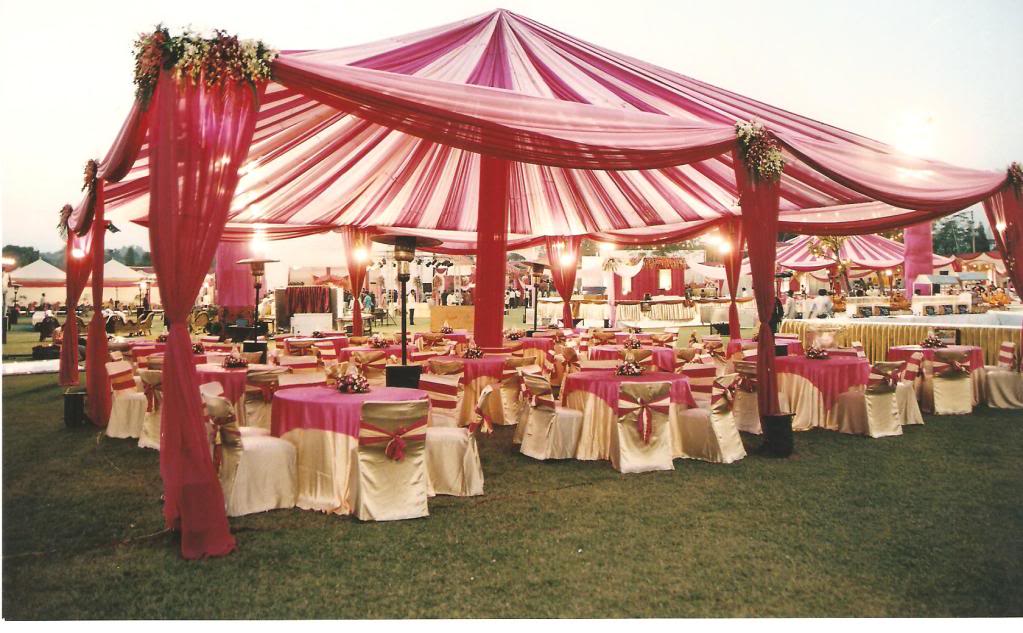This image captures an elegant outdoor wedding or celebration beneath a grand red and white striped tent, reminiscent of a festival canopy. The tent is adorned with drapes cascading down from the posts, accented by clusters of flowers at the top of the columns. Underneath this elaborate canopy, situated on a lush grassy field, are approximately 12 to 15 dining tables. Each table is elegantly decorated with tablecloths that transition from a maroon-pinkish hue at the top to cream at the bottom. The chairs around the tables are draped in matching cream and gold fabric, with bows tied at the back in a red and cream, pinkish-red shade. The scene is illuminated by white lights strung around the tent, enhancing the festive atmosphere. In the distance, additional similar structures can be seen, with people meandering about, suggesting the event is about to commence. The overall ambiance is one of meticulous detail and sophisticated celebration, set against a beautifully serene backdrop.